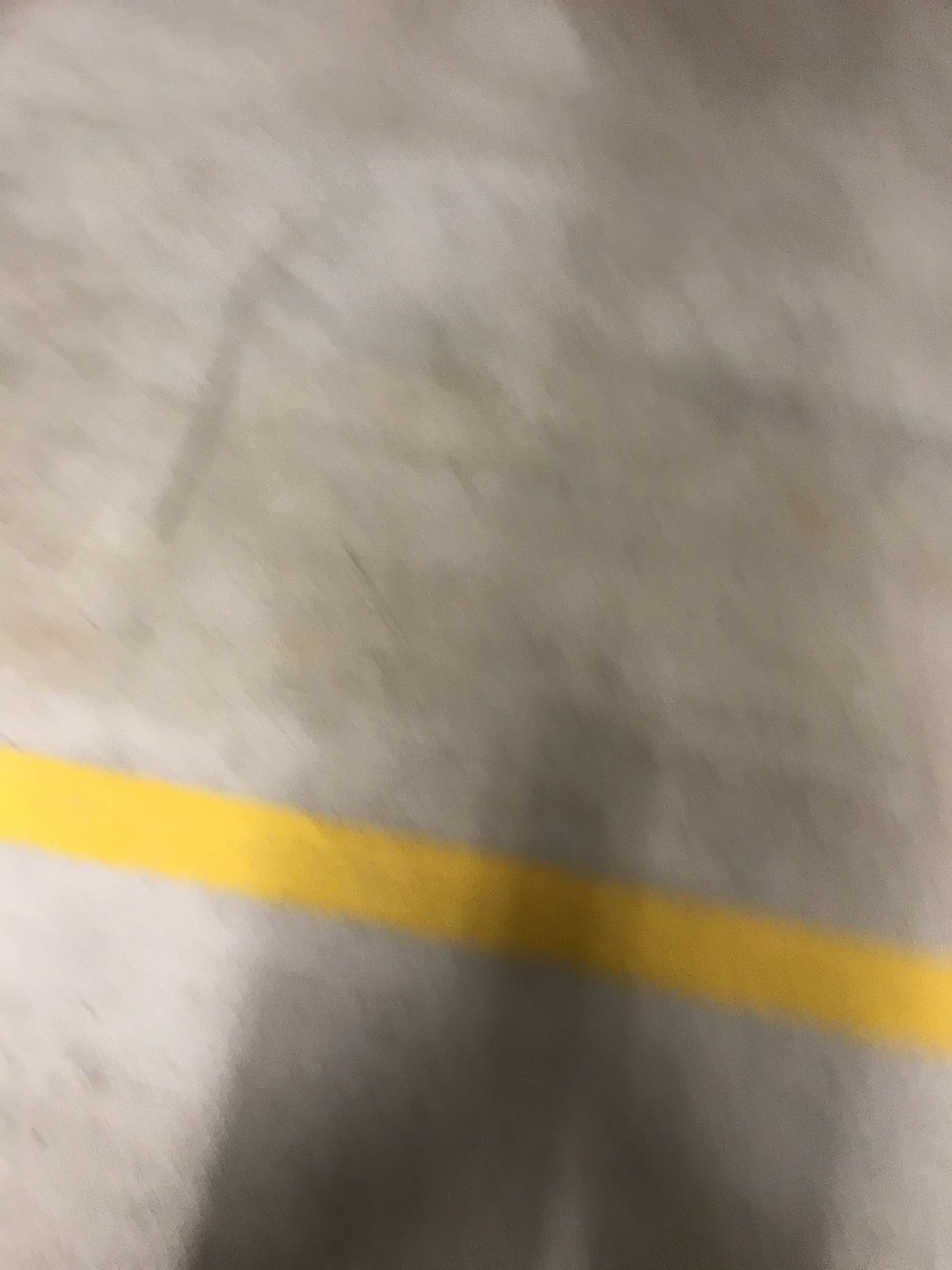The image depicts a vertically rectangular, blurry, and underexposed scene that seems to capture a section of pavement. The predominant hue is a dark to light gray, suggesting an inconsistent texture that resembles a roughly surfaced road. Extending from the lower right corner diagonally to just below the center of the left side is a thin yellow or occasionally perceived as white line, painted onto the pavement, standing out amidst the gray background. Notably, there is a shadow, presumably from the photographer, cast onto the pavement. This shadow appears centrally aligned with the yellow line, with the legs of the shadow being distinctly clearer than the upper body, which becomes increasingly obscure upwards. The lighting indicates that the source might be positioned behind the person taking the picture.